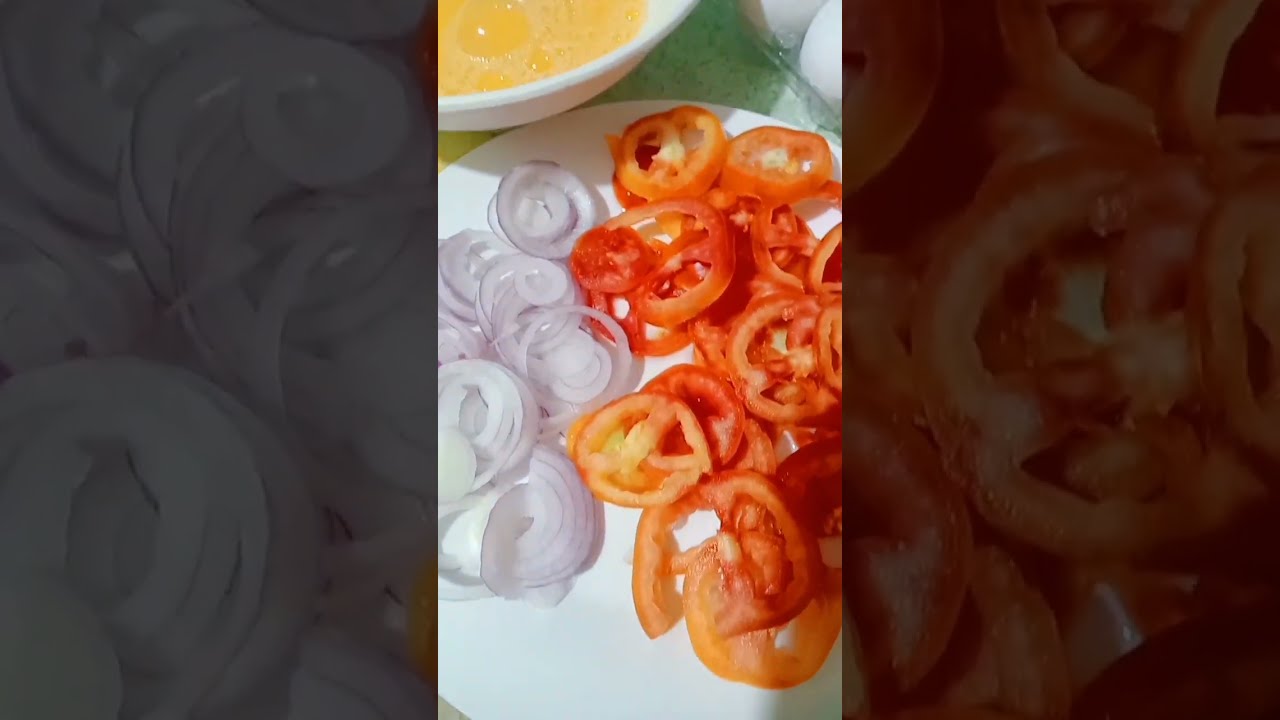The horizontal rectangular image features a central vertical photograph framed by grayed-out areas on either side. The clear central photograph captures a white plate of food from a top-down perspective. On the left half of the plate, there are circles of sliced red onion, while the right half is occupied by irregularly cut, somewhat unappetizing red tomato slices. The plate lies on a white background, potentially a table or countertop. Above the plate, near its upper corner, a bowl with yellow liquid, likely melted butter, is partially visible. Additionally, broken eggshells and unused eggs appear to be placed near the edge of the frame, but no cooking instruments are present.